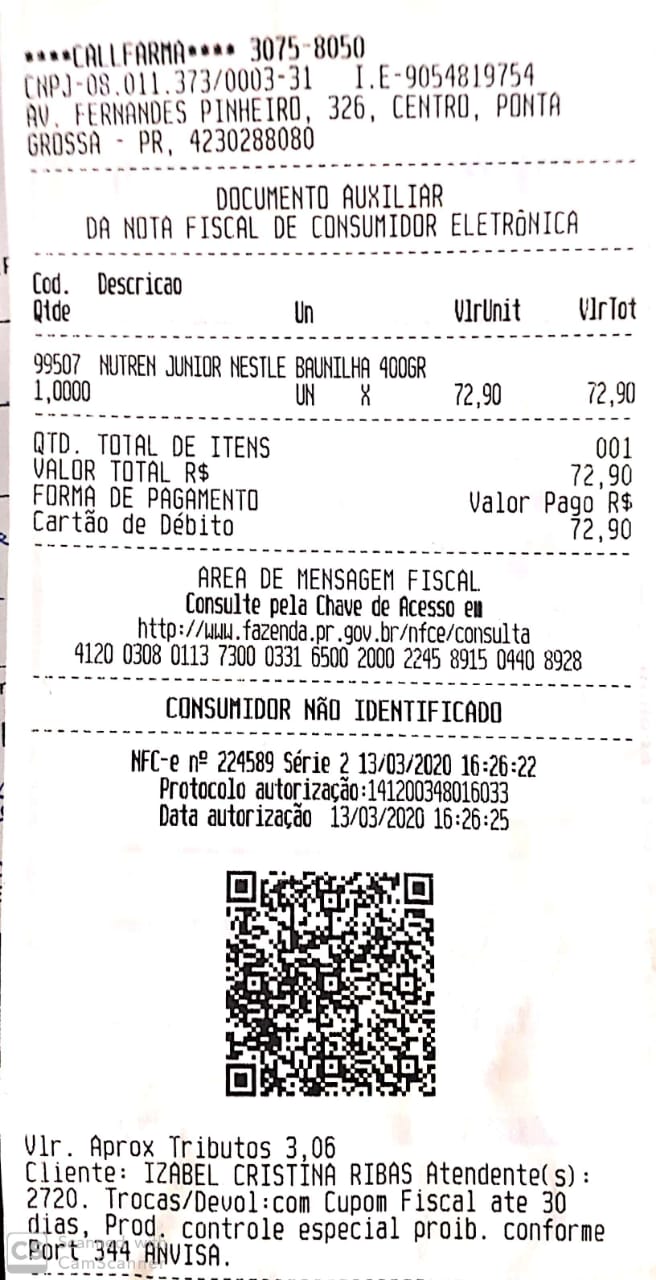In this image, a white receipt with black print is displayed against a white background. The top of the receipt features the text "California" and "Centro Ponta Grossa," indicating a likely location or establishment name. The receipt includes a barcode and a quick response (QR) code for scanning. The list of purchased items is detailed in Spanish, making it hard to interpret for non-Spanish speakers. At the bottom, the total amount of $72.90 is indicated, presumably paid via a credit card.